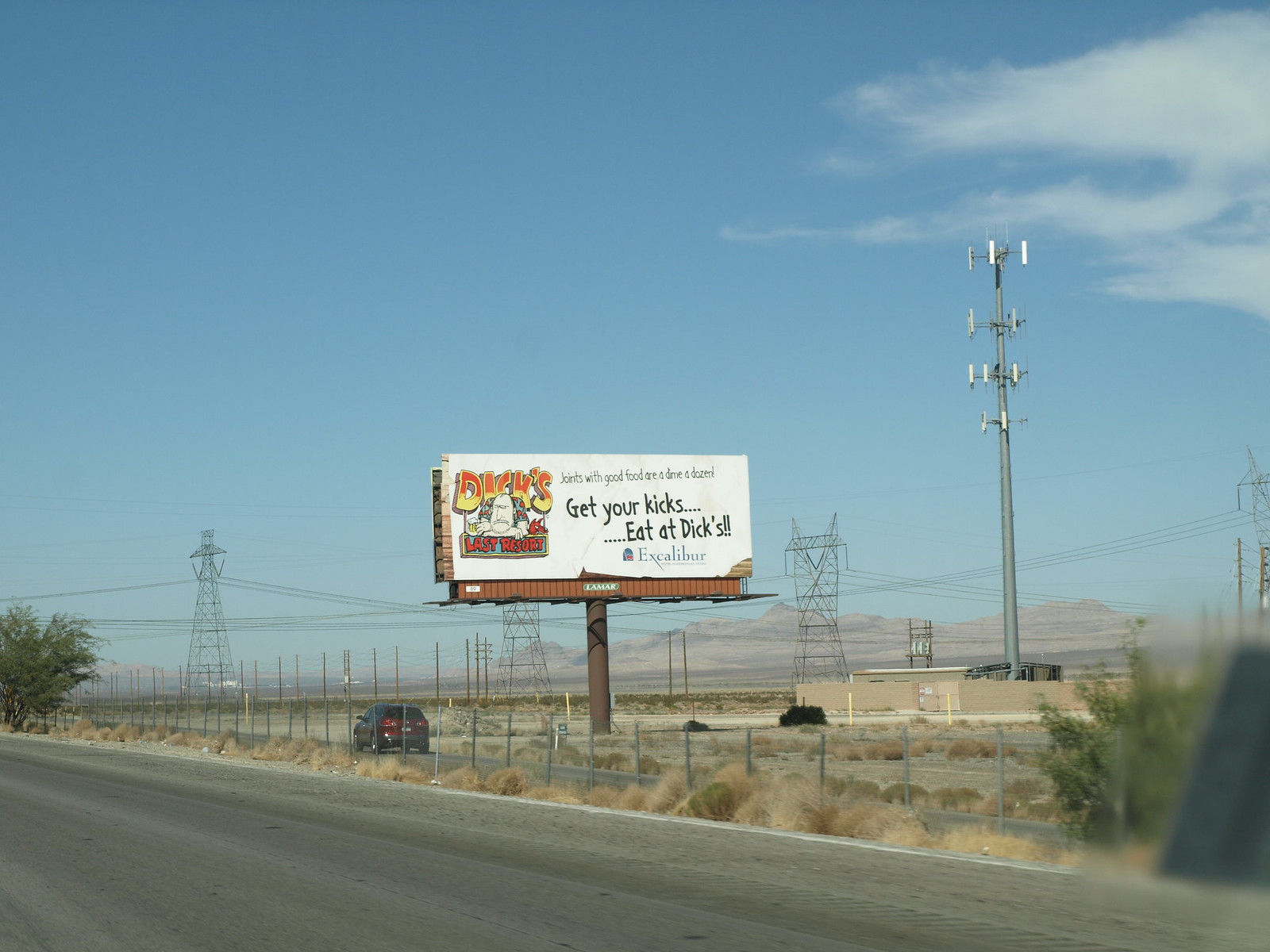The photograph captures a scene from a moving car, evident by a small sticker on the windshield's right corner. It depicts a maroon SUV driving along a gray road, paralleled by another road separated by a tall, gray metal fence. Dominating the scene is a large billboard mounted on a dark brown, cylindrical pole with a white background. The billboard features an advertisement for a restaurant called Dick's, stating in red and black text: "Joints with good food are a dime a dozen. Get your kids, eat at Dick's. Excalibur." A bald man peeks over a smaller sign that reads "Last Resort." In the background, a sprawling landscape unfolds with large radio towers stretching across the scene, set against a distant light gray or light brown mountain range. The sky above is blue, adorned with wisps of white clouds in the right corner. Verdant elements punctuate the arid terrain, with a dark green tree visible in the left corner and a bush close to the car. This detailed snapshot emphasizes the contrast between the industrial elements, such as the black, thin power lines and radio towers, and the natural environment.